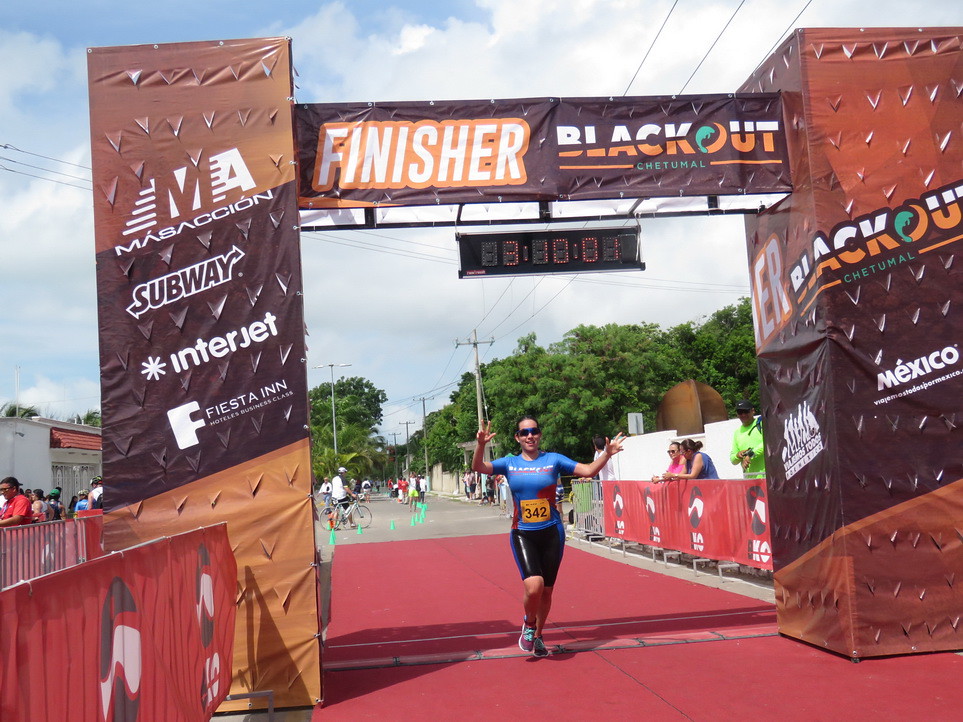The photograph captures the dramatic moment at the finish line of a marathon, adorned prominently with a red carpet. Metal pillars made of scaffolding wrapped in alternating light and dark brown banners flank the finish line, supporting a sign board overhead. This sign board, also constructed from scaffolding, features a large LED timer displaying "31:00:01" in orange digits, alongside the emblazoned text "FINISHER BLACKOUT CHETUMAL," indicating both the culmination of the race and its sponsors.

A woman, smiling and triumphant, is crossing the finish line. She's wearing a blue shirt with red markings, black knee-length yoga pants, and vibrant red and green athletic shoes. Her bib number "342" is prominently displayed on her stomach. The left column showcases multiple sponsor logos: Massachion, Subway, Interjet, and Fiesta Inn, while similar sponsor banners line the course on both sides. Spectators, including some women, watch from behind the barriers, adding to the lively and bustling atmosphere of this sunlit event.